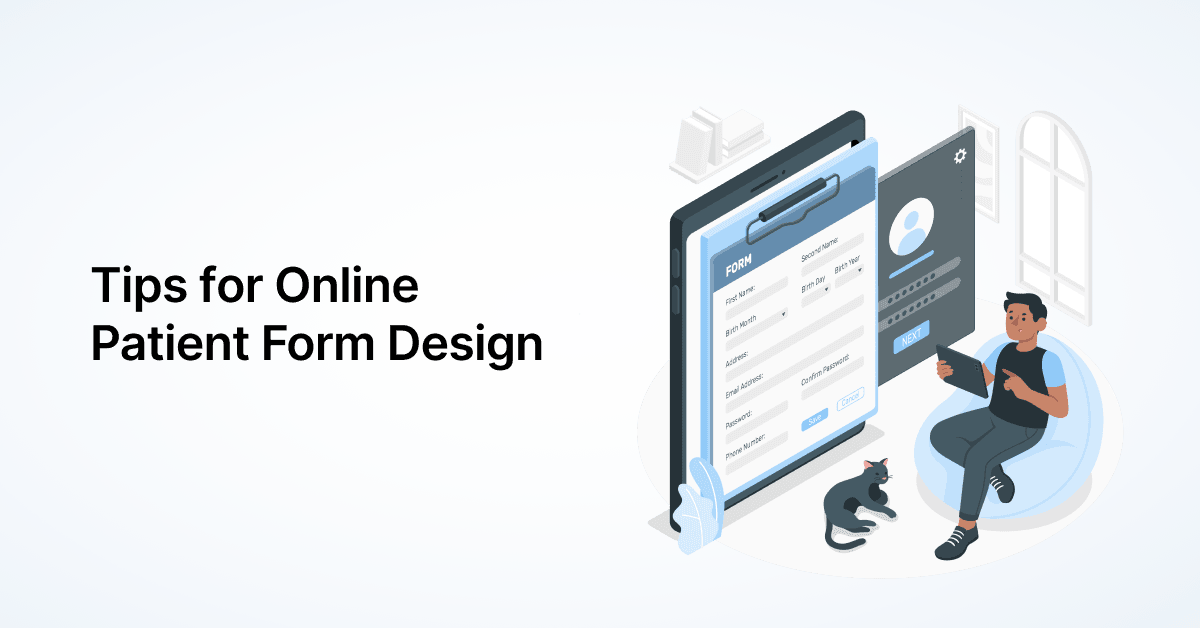The image features a crisp white background, with the text "Tips for Online Patient Form Design" prominently displayed in black Arial font on the left side. On the right side, there is a detailed, computer-generated color illustration. The central element is a large, visually emphasized black tablet screen displaying an online form with a blue banner and several text boxes underneath. Adjacent to this screen is a smaller login interface featuring a default user profile icon, fields for username and password, and a blue "Next" button.

In the foreground, a man with brown skin and black hair is seated in a blue beanbag chair. He is wearing a black vest with blue sleeves, gray pants, and black shoes, holding a tablet in his right hand, presumably engaging with the form. At his feet lies a black and gray cat, lounging tranquilly.

The background includes several architectural elements, including a couple of arched windows and a faint depiction of a bookshelf. The illustration merges a modern, digital experience with cozy, relatable elements, effectively emphasizing the tips for designing patient forms in an online setting.